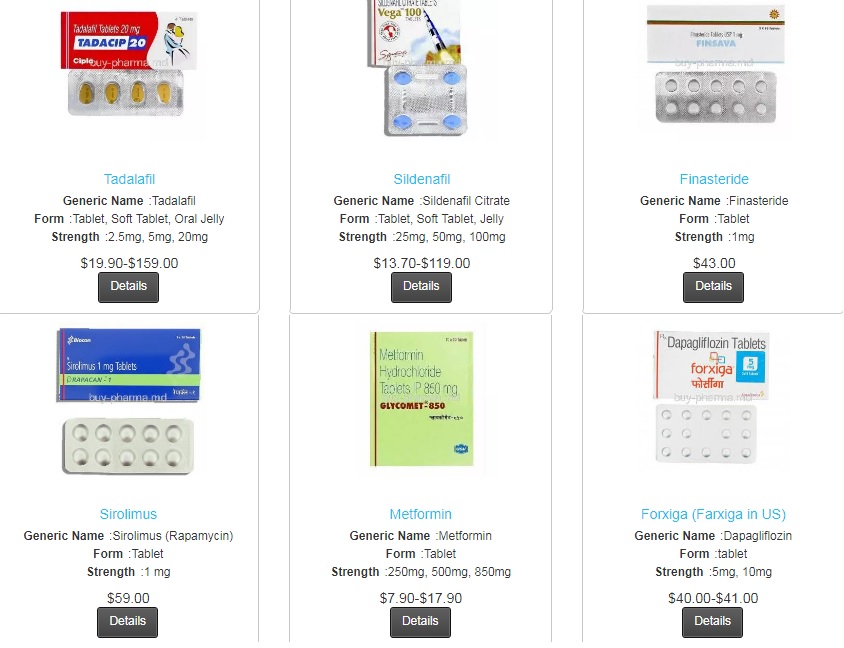**Detailed Caption:**

The vertical image showcases an online store interface displaying pharmaceutical products in a neatly organized grid. The layout consists of two rows, each containing three items, making a total of six products available for browsing. Each product listing includes an image, product name, generic name, form, strength, price, and a button for additional details.

**Top Row:**
1. **Tadalafil**:
   - **Generic Name:** Tadalafil
   - **Form:** Tablet, Soft Tablet, Oral Jelly
   - **Strengths:** 2.5 mg, 5 mg, 20 mg
   - **Price:** $19.90 to $159 
   - A gray button labeled "Details" in white text is available for more information.
  
2. **Sildenafil**:
   - **Generic Name:** Sildenafil Citrate
   - **Form:** Tablet, Soft Tablet, Oral Jelly
   - **Strengths:** 25 mg, 50 mg, 100 mg
   - **Price:** $13.70 to $119 
   - A "Details" button in gray and white is provided.

3. **Finasteride**:
   - **Generic Name:** Finasteride
   - **Form:** Tablet
   - **Strength:** 1 mg
   - **Price:** $43 
   - Includes a button labeled "Details" for further options.

**Bottom Row:**
All these items follow the same format as the top row with images at the top, names in blue beneath the images, and important details such as the generic name, form, and strength in bold black text. The prices are listed in a lighter black text, and each listing has a "Details" button for more information.

This organized and informative layout enables users to easily browse medications, compare options, and access detailed descriptions, helping them make informed purchasing decisions.